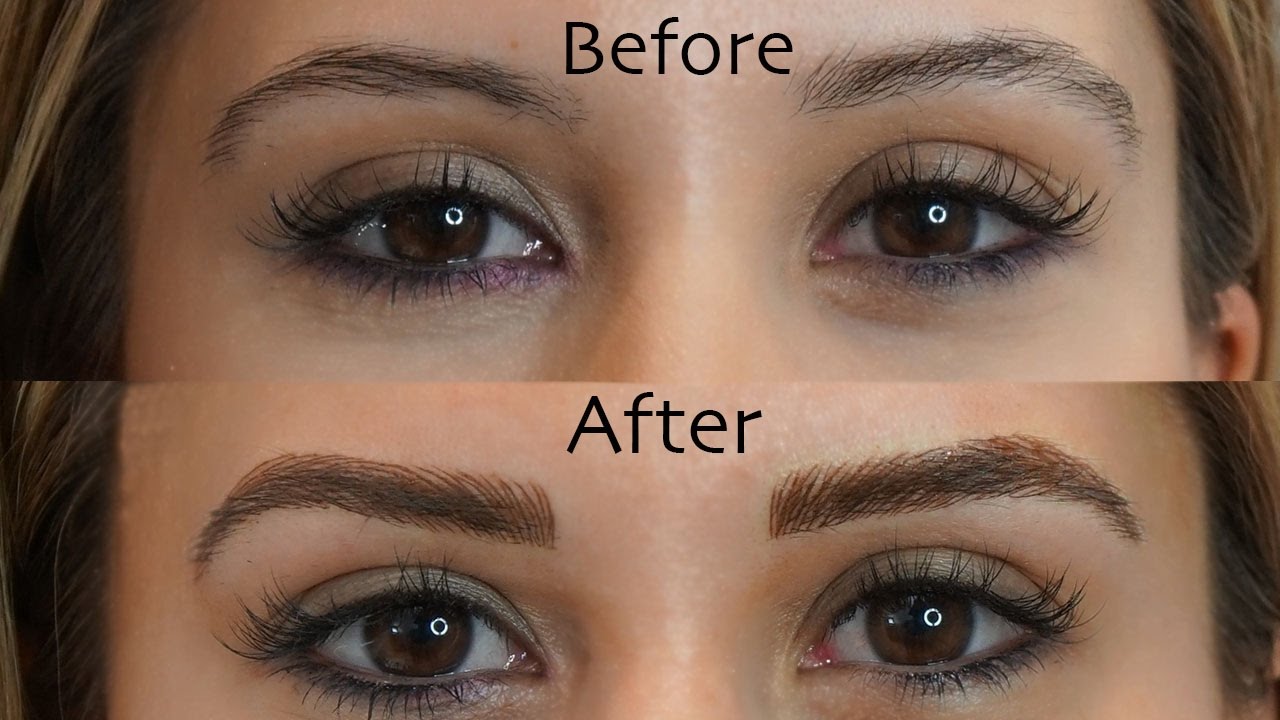This is a before-and-after image, with the before photo on top and the after photo on the bottom. Both images focus closely on a woman's eyes, extending from just above the tip of her nose to just above her eyebrows. The woman has brown hair, light skin, and brown, almond-shaped eyes with black eyelashes. 

In the before image, her eyebrows appear slightly lighter and less defined. The after image showcases subtly thicker, more evenly shaped eyebrows that follow the common aesthetic trends. The refined eyebrow work highlights a slight difference in makeup application around the eyes, making them appear more open. Despite the subtle changes, the overall lighting and the reflected light source in her eyes remain consistent between the two photos, emphasizing the minor enhancements rather than drastic alterations.